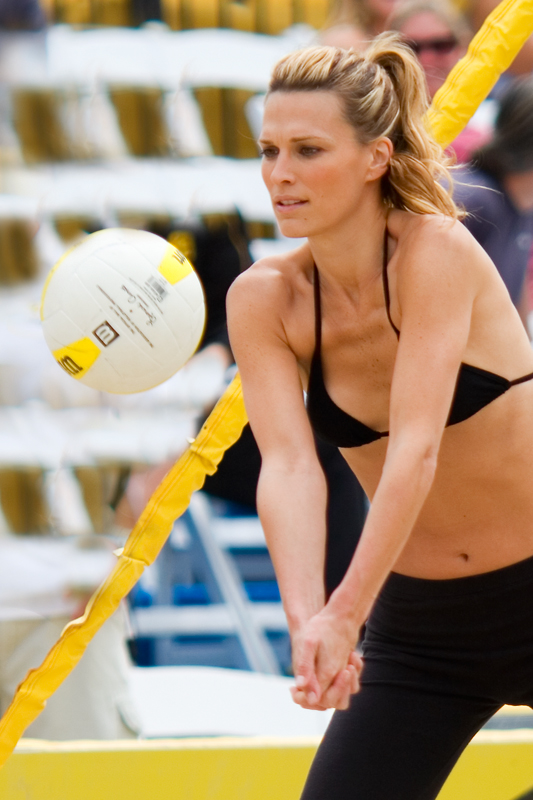In this action-packed outdoor volleyball game, a tall and toned athletic woman with her blonde hair tied back into a ponytail, where the roots reveal a dark brown hue, is captured mid-play. She is dressed in a black bikini top and long black yoga pants, showcasing her tan complexion. With a focused and serious expression, her mouth slightly open, and her eyebrows almost out of frame, she positions her arms into a triangle, hands clasped together, ready to volley a white volleyball detailed with yellow stripes and the brand "Wilson" prominently displayed. In the blurred background, spectators sit in bleachers, hinting at the intensity of the game. The white net in front of her, designed with a pattern of little squares, underscores the sporting context while an older woman in black sunglasses appears faintly in the distance.